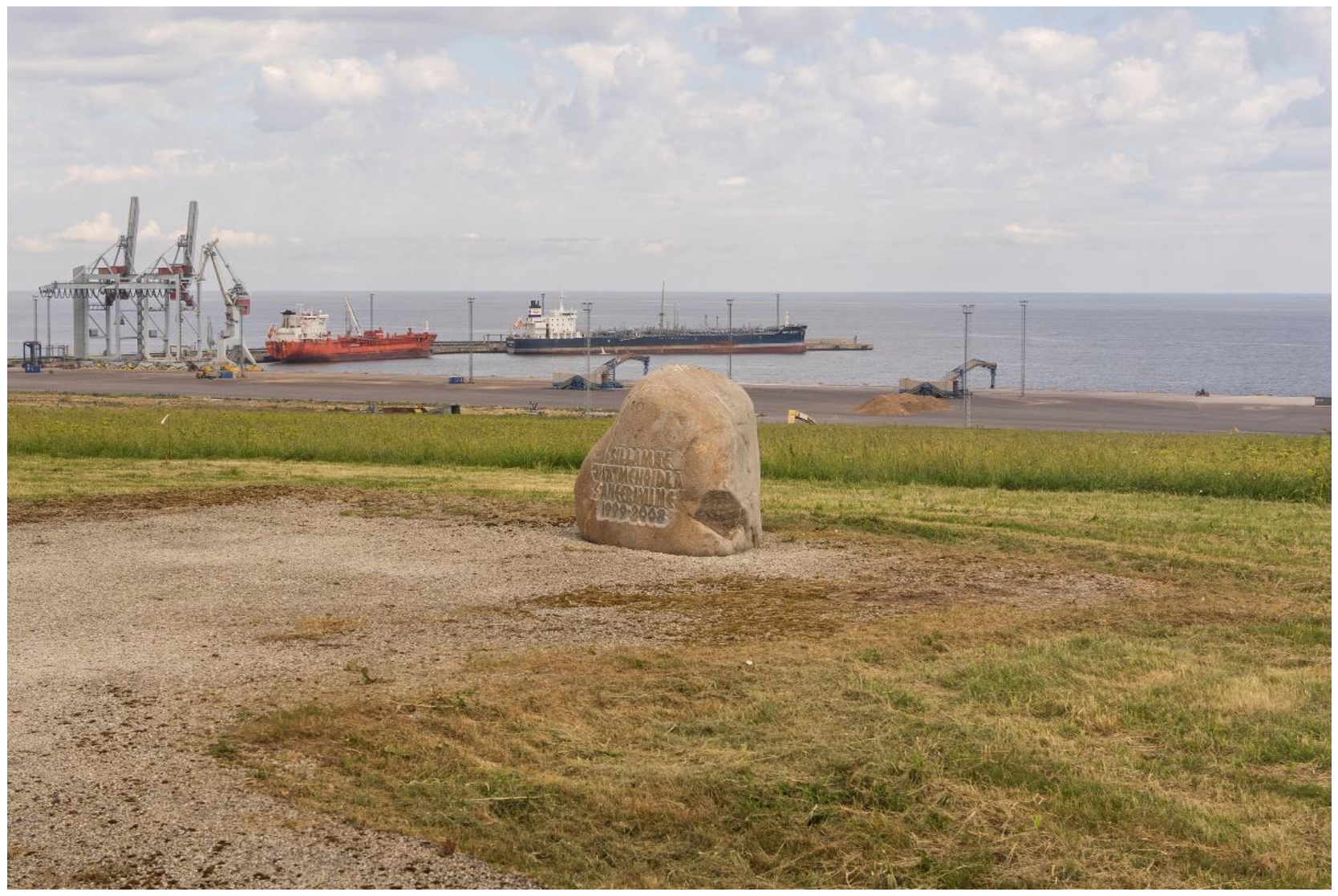In this photograph, we see a prominent beige stone marker set on a sparse patch of grass and soil near a waterfront. The marker features an inscription, possibly reading "Sillamack," followed by several words and the dates "1999 to 2008." The setting around the marker seems quite plain, contrasting with the industrial backdrop. Behind the stone, there's a busy seaport, with large ships docked near industrial machinery, possibly involved in drilling operations. The waterfront scene is accentuated by a light blue sky dotted with white clouds. This solemn marker, clearly a monument, is juxtaposed against the bustling activity of the industrial port, emphasizing its presence amidst the utilitarian surroundings.